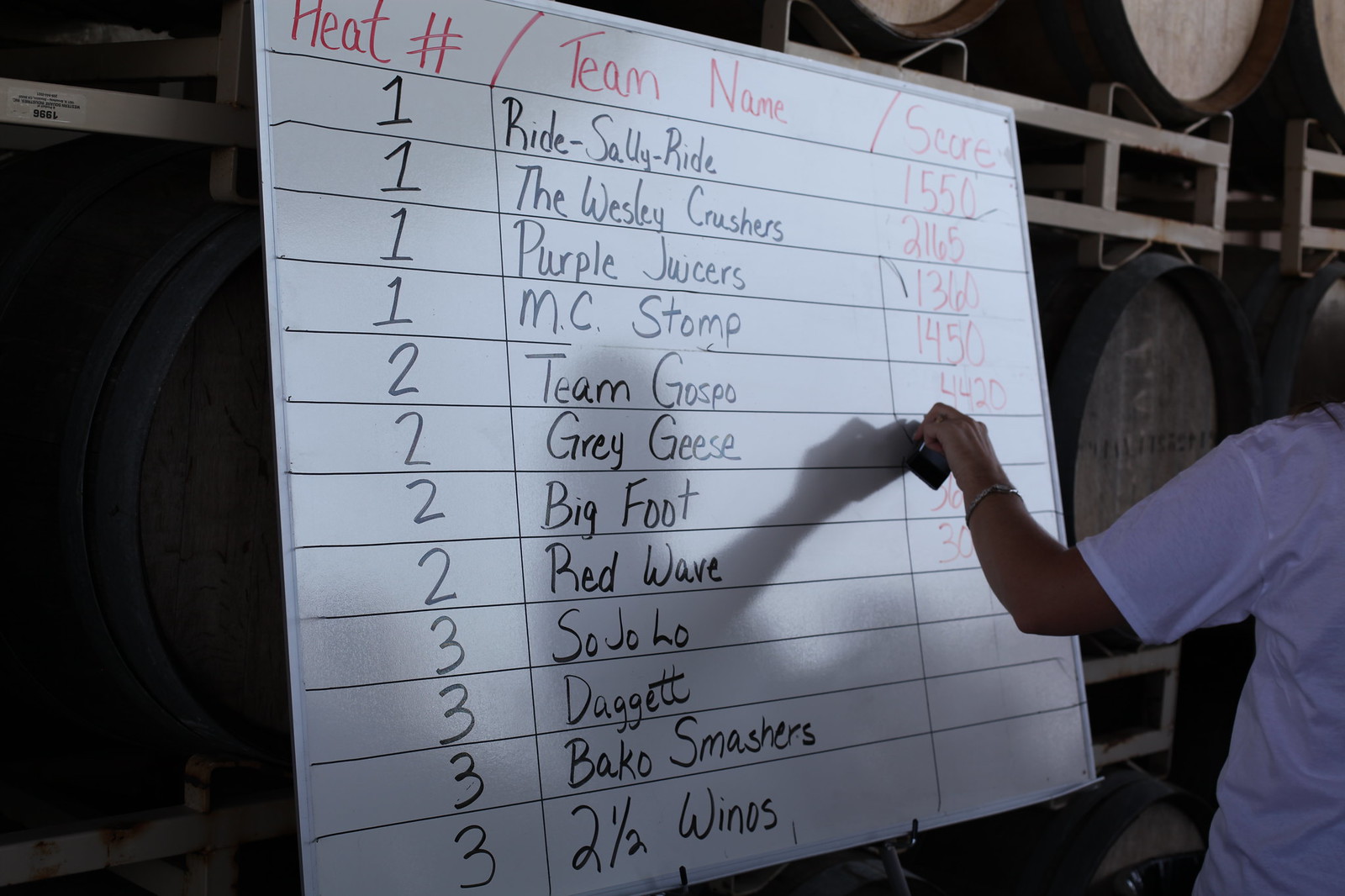In the image, the setting appears to be indoors, during some kind of competition. Dominating the center is a large sign divided into three sections labeled "HEAT NUMBER," "TEAM NAME," and "SCORE," written in red marker. The teams listed include Ride Sally Ride, The Wesley Crushers, Purple Juicers, MC Stomp, Team Gospo, Grey Geese, Bigfoot, Red Wave, Sojo Low, Daggett, Backhoe Smashers, and Winos. Scores for some teams are visible: Ride Sally Ride has a score of 1550, The Wesley Crushers 2165, Purple Juicers 1360, MC Stomp 1450, and Team Gospo 4420. Grey Geese's score is partially erased by a person holding an eraser on the right side of the image, and the scores for Bigfoot, Red Wave, Sojo Low, Daggett, and Winos are not visible. In the background, a series of barrels are stacked on shelves. The colors featured in the image include black, white, red, gray, off-white, and brown.